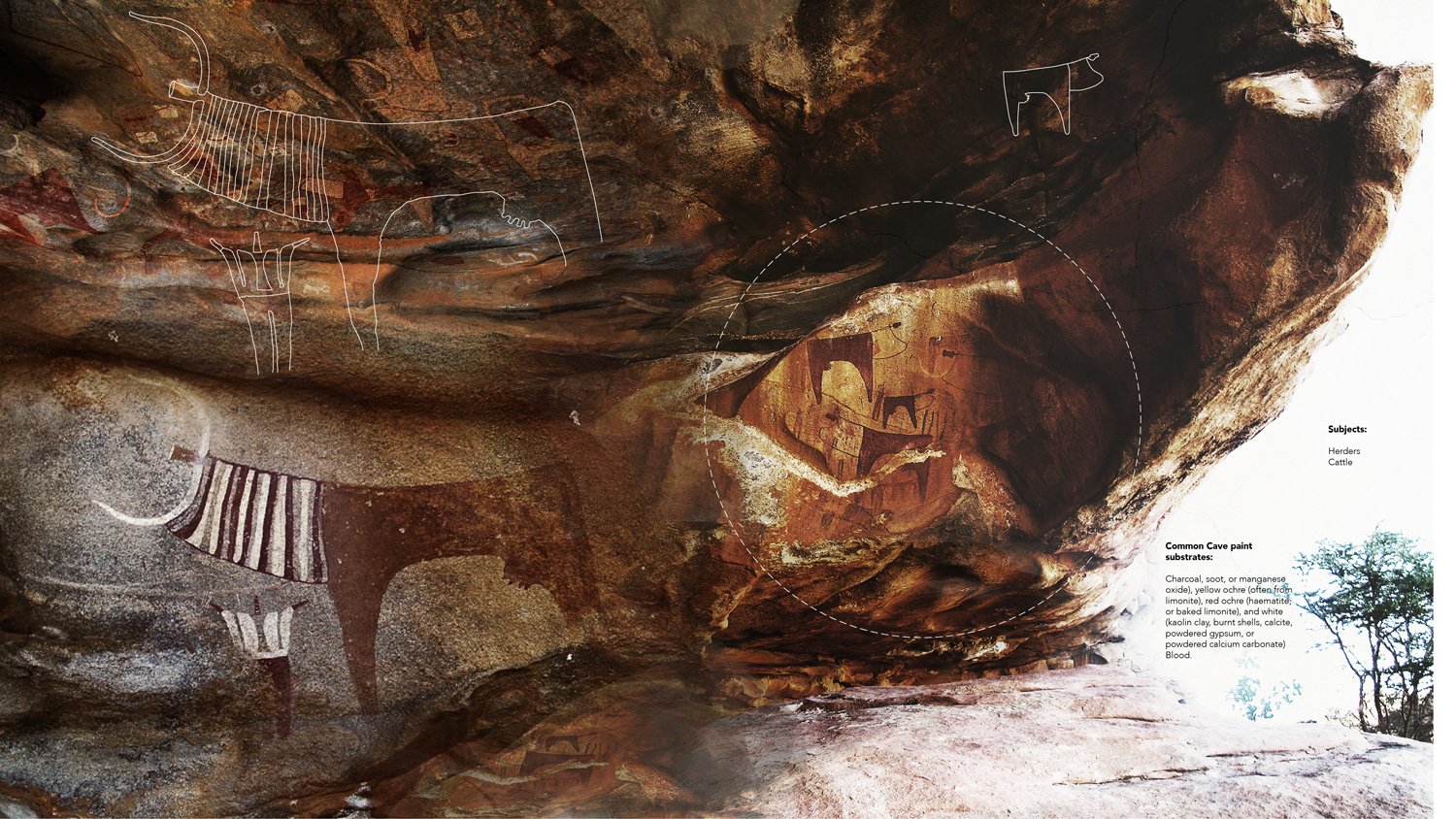The image depicts a large rock surface, potentially inside a cave, adorned with ancient pictographs. At the center, a long-faded drawing of a white animal, likely created by early humans, is accompanied by a face etched to its right. Above, a reddish-brown bowl-stenciled outline is visible, matching an actual painted bowl just below it. This bowl features white stripes and legs detailed in both white and brown hues. The top left corner of the image contains a red-tinted, mesa-like structure with legs, and another animal drawing that appears bovine, with distinctive horn-like features and an udder. A dotted line circumscribes this upper section, highlighting these archaic works, reminiscent of textbook illustrations used to delineate and emphasize key elements.